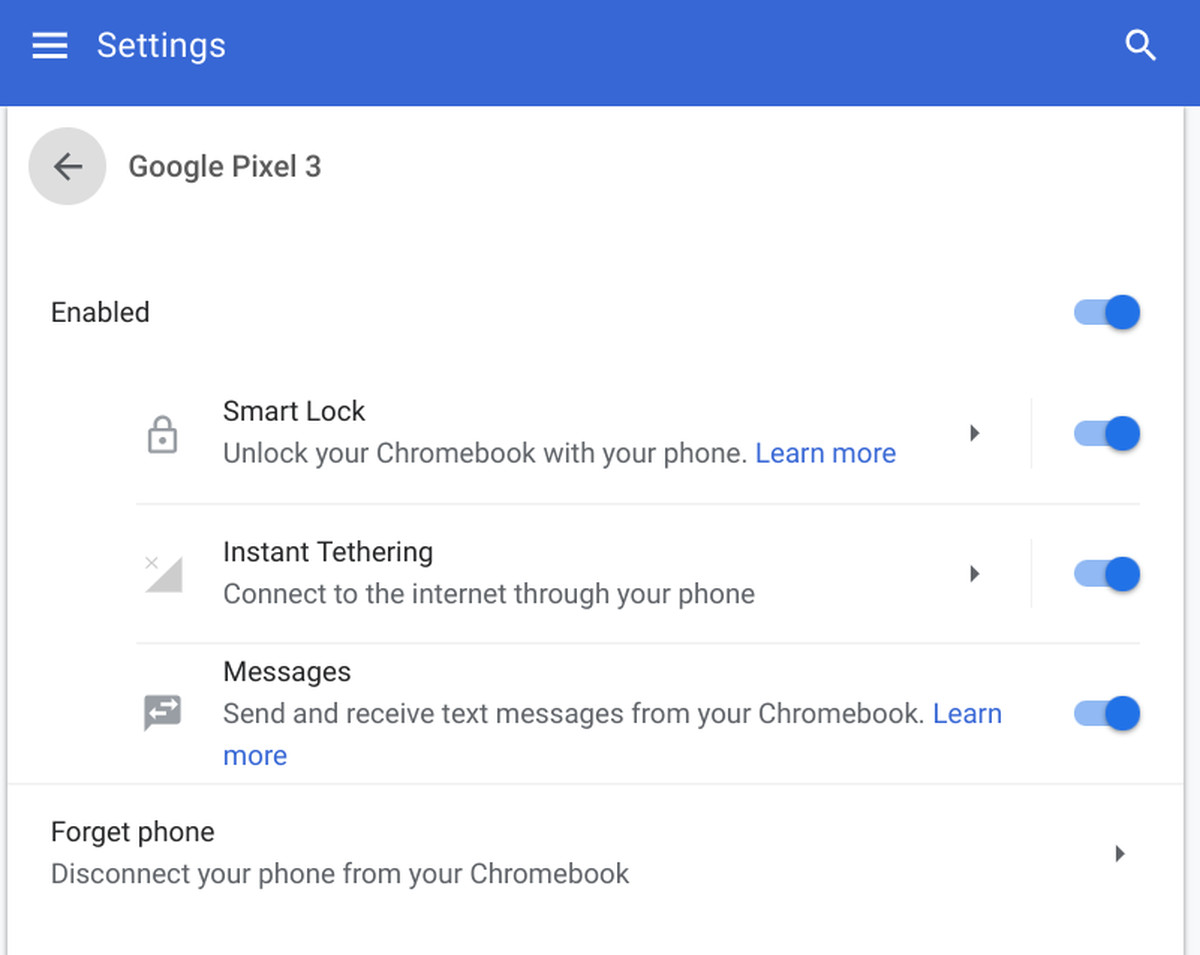**Caption:**

Detailed view of the settings page for Google Pixel 3, showing various enabled features.

At the top of the screen, there is a blue-bordered header that includes a hamburger menu icon on the left, followed by the word "Settings." To the far right of the header, there is a search icon.

Below the header, within the main white body of the page, a left-facing arrow is labeled "Google Pixel 3." Underneath this title, the status "Enabled" is displayed, accompanied by buttons to either enable or disable various features.

1. **Smart Lock:**
   - **Icon:** Lock
   - **Description:** “Unlock your Chromebook with your phone.”
   - **Action:** Learn more
   - **Status:** Enabled

2. **Instant Tethering:**
   - **Icon Description:** Connect to the internet through your phone.
   - **Status:** Enabled

3. **Messages:**
   - **Description:** Allow sending and receiving text messages from your Chromebook.
   - **Action:** Learn more
   - **Status:** Enabled

Finally, there is an option labeled “Forget phone,” which provides the ability to disconnect your phone from the Chromebook. This option is accompanied by a right-facing arrow.

In summary, this settings page for the Google Pixel 3 allows users to manage and enable features such as Smart Lock, Instant Tethering, and Messages, with all options currently enabled. Users also have the option to disconnect their phone from the Chromebook.